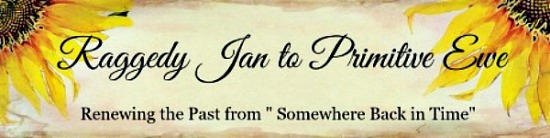The image features a large horizontal banner set against a predominantly white background with a yellowish tint at the center. On either upper corner, there are partially visible sunflowers, each showing about a quarter of their centers surrounded by vibrant yellow petals. The centerpiece of this banner is black script text that reads, "Raggedy Jan to Primitive Eve," signifying a journey or transformation. Below this, simpler black text in a straightforward font states, "Renewing the past from 'somewhere back in time.'" The banner fills the entire frame, devoid of any other objects, suggesting a decorative style likely intended for a website or similar digital platform. The color palette includes tan, black, yellow, orange, red, and gray, contributing to the overall rustic and nostalgic aesthetic.